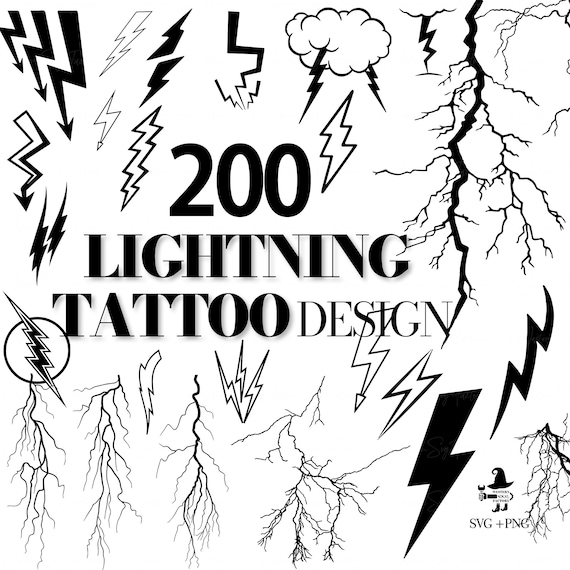This image is a black and white chart or poster, typically found in a tattoo parlor, illustrating various lightning bolt designs for tattoo options. Set against a white background, the poster prominently features the text "200 Lightning Tattoo Designs" in the middle, with the word "Designs" appearing in a skinnier and somewhat harder-to-see font. The fonts for "200" and "Lightning Tattoo" are differently styled, with "200" in a standard font and "Lightning Tattoo" in a more varied and stylized font.

The poster showcases approximately 15 visible examples of lightning bolt designs in different styles and configurations. Some designs depict multiple streaks of lightning, while others feature clouds with lightning bolts descending from them. There are bold, solid lightning bolts, and some incorporate arrows at the end. Others resemble veins or a part of a lightning storm with intricate zigzag patterns. In the upper left-hand corner, there is a trio of lightning bolts zigzagging to the right and left, ending in arrows. 

In the lower right-hand corner, there is text indicating "SVG and PNG" along with what appears to be a company logo, suggesting these designs might be available for digital purchase, possibly from an online store such as Etsy for use with a Cricut machine.